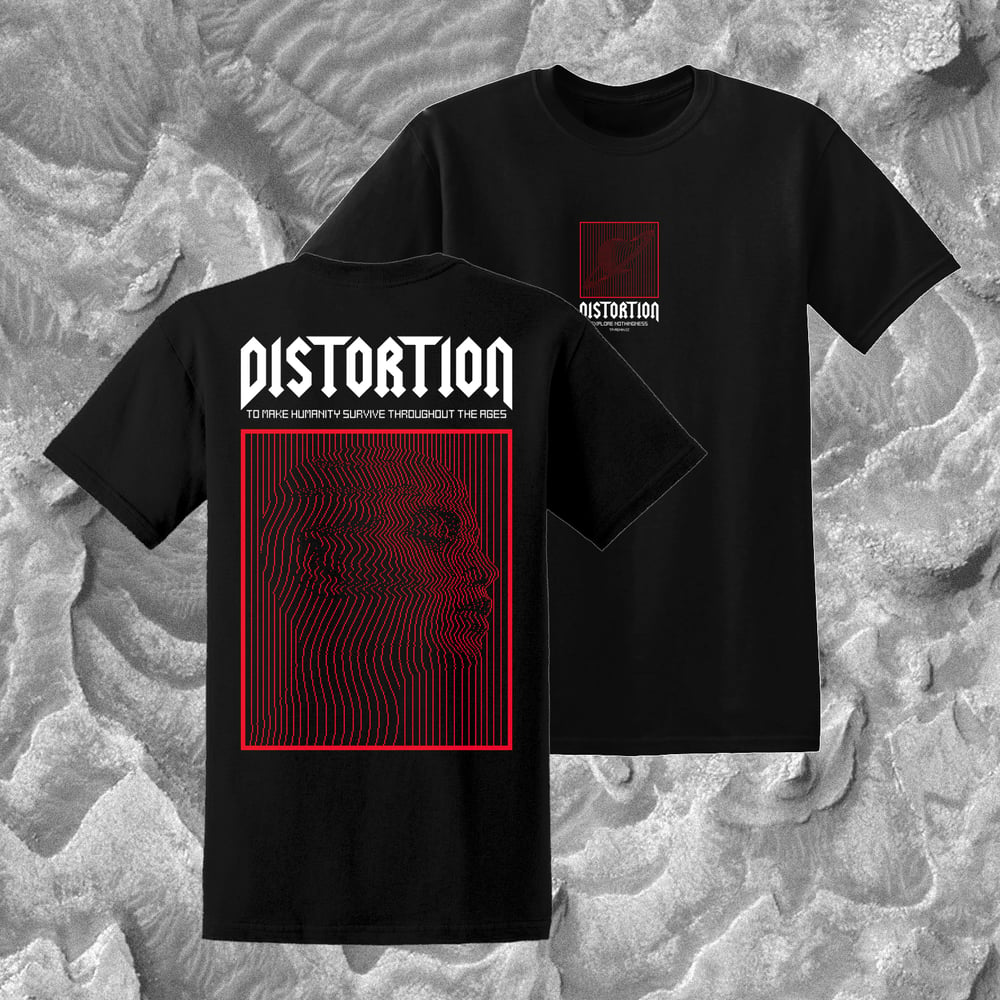This image features two black t-shirts set against a textured, variegated gray background that resembles a stone surface. Each shirt displays a bold, white capitalized word "DISTORTION" at the top. Below this, one shirt features the slogan "to make humanity survive throughout the ages" in white text. Both shirts showcase a red-bordered graphic of a bald human face shown in profile, facing right, with closed eyes and lips. The face is created with vertical red lines against the black fabric of the shirt, giving it an intricate, layered design. The graphic on one shirt appears larger and is placed centrally, while the other shirt exhibits a smaller version of the same image. This detailed and artistically layered design gives the t-shirts a striking visual appeal, suggesting they are likely advertised for sale.